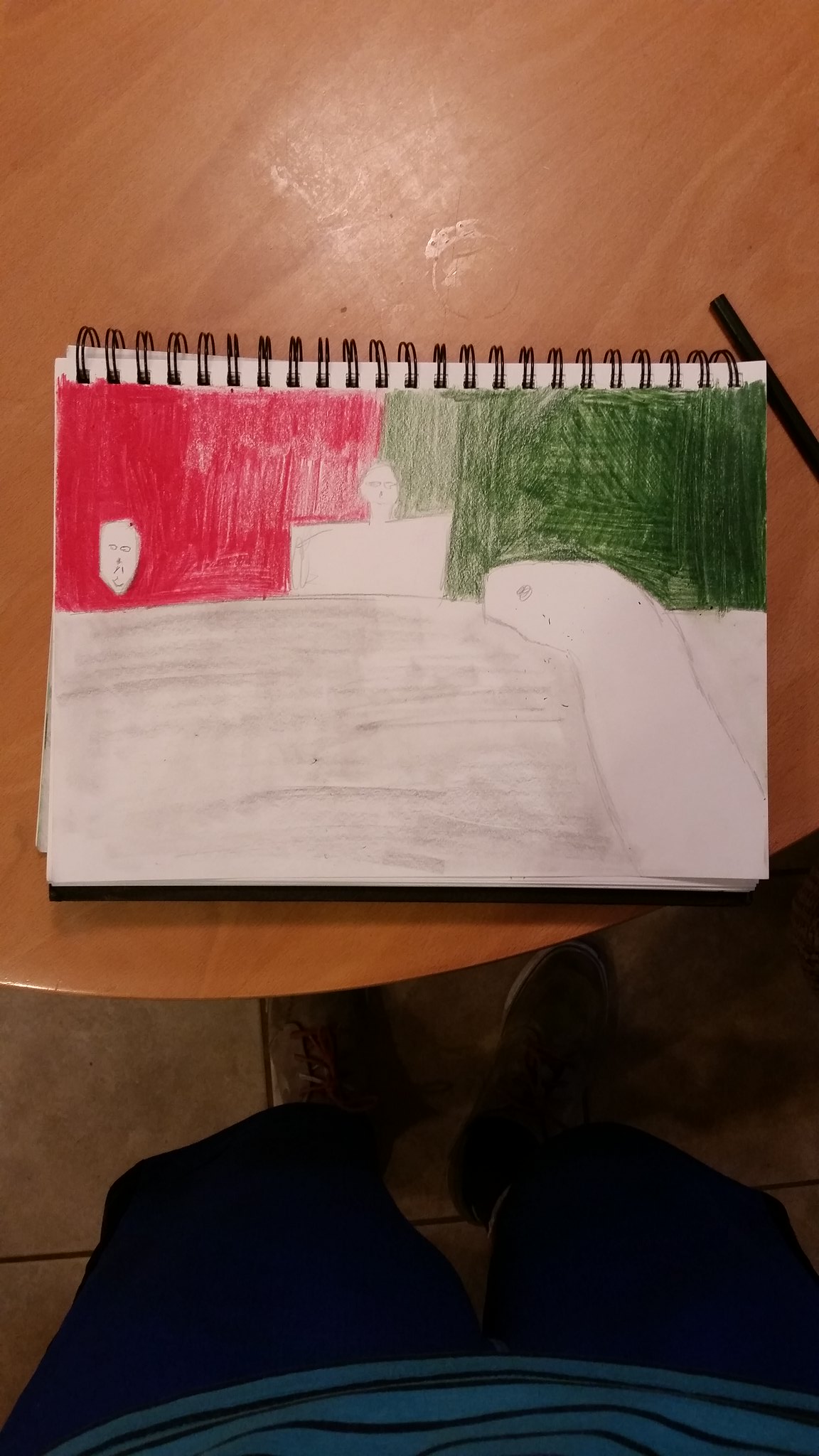Caption: 

A bird's-eye view captures a person standing on a tile floor, identifiable by their black shoes, black pants, and blue shirt with black stripes. Positioned directly above a wooden table, the individual is photographing their drawing pad which rests there, alongside a pen. The drawing pad displays a meticulously sketched scene featuring a dinosaur or reptile emerging from a body of water. Behind this prehistoric creature stands a person on the shore, next to a building. The bottom half of the drawing is shaded with pencil to simulate water, while the top half is divided into two sections—one side adorned with green hues and the other with red, adding a dynamic and colorful contrast to the scene.